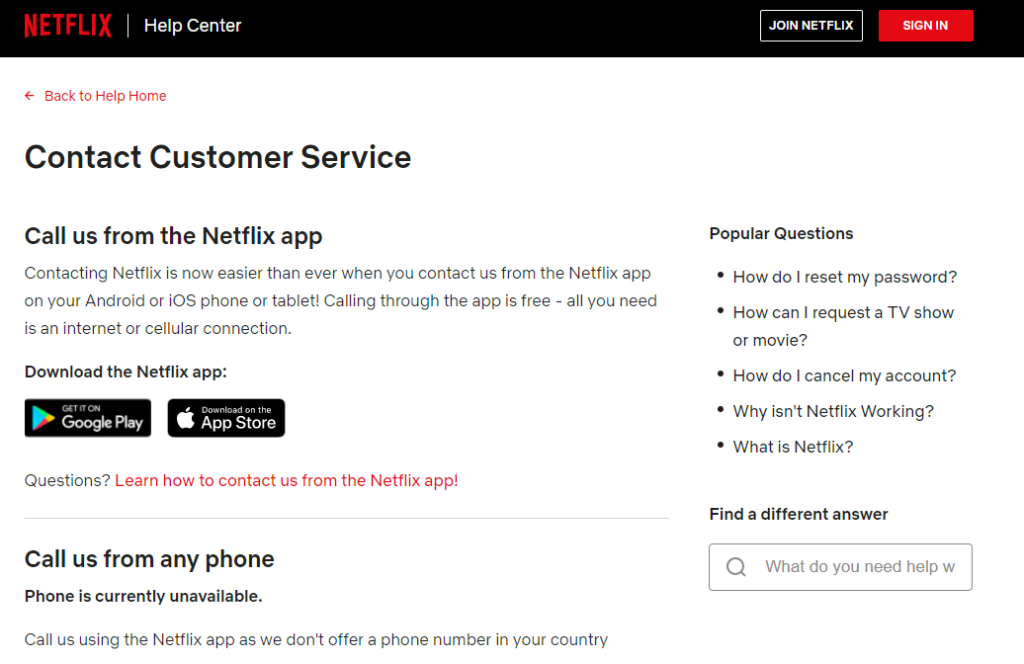Screenshot of a Netflix Help Center page displayed in a horizontal layout. At the top, a thin black bar features the red Netflix logo on the left and "Help Center" in white text. On the right side, there are two buttons: a white-bordered button labeled "Join Netflix" in white text, and a red button labeled "Sign in" in white text.

Below the black bar, the rest of the page has a white background. At the top, there is a red link labeled "Back to Help Home." Underneath, a black header reads "Contact Customer Service." The main text explains how to call Netflix from the app: "Contacting Netflix is now easier than ever when you contact us from the Netflix app on your Android or iOS phone or tablet. Calling through the app is free. All you need is an internet or cellular connection. Download the Netflix app." Beneath this text, there are two black buttons: "Get it on Google Play" and "Download on the App Store."

Following this, a section titled "Questions" instructs users on how to contact Netflix from the app. At the very bottom, another notice reads: "Call us from any phone. Phone is currently unavailable. Call us using the Netflix app as we don't offer a phone number in your country."

On the right-hand side, there is a list of popular questions in bullet points:
- How do I reset my password?
- How can I request a TV show or movie?
- How do I cancel my account?
- Why isn't Netflix working?
- What is Netflix?